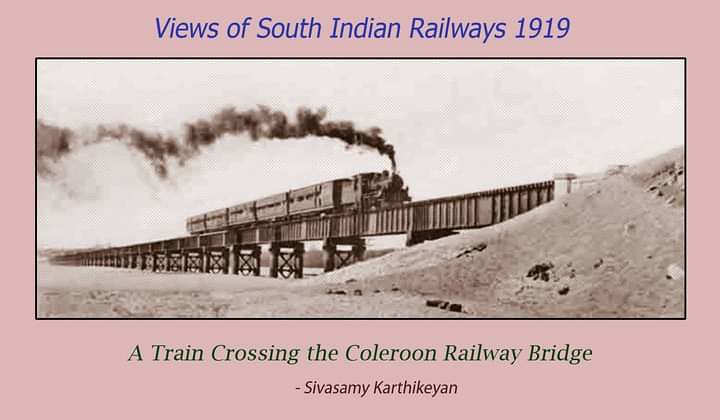This is an image with a very light purple background, possibly taken from a book or the front cover of a postcard. The layout is horizontal with a rectangular shape. At the top center, in italicized blue sans serif font, the text reads "Views of South Indian Railways 1919." Below the title is a black-bordered photograph featuring a sepia-toned or black-and-white train crossing a metal bridge known as the Kholroon Railway Bridge. The train has five cars trailing behind the engine, which emits a long plume of black smoke. On the right side of the photograph, there is a hill that the bridge connects to. Centered beneath the image, in green serif font, it states "A train crossing the Kholroon Railway Bridge," followed by the photographer's credit in small font: "Sivasamy Karthikeyan."